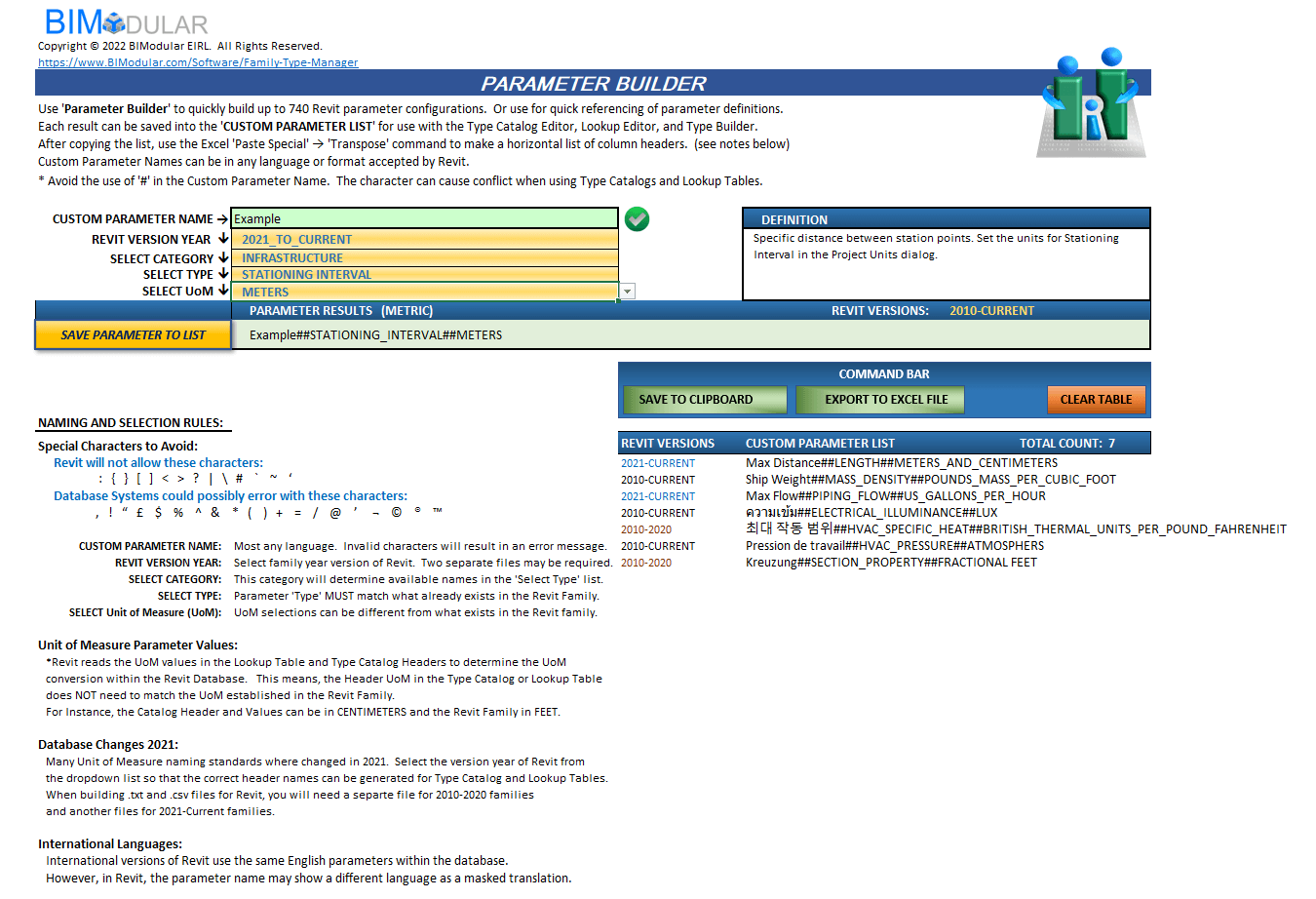This image, sourced from the BIModular website, displays the Parameter Builder interface. At the top, the header reads "Parameter Builder," accompanied by a copyright notice: "© 2022 BIModular EIRL, all rights reserved." The official website URL, bimodular.com, is also prominently displayed.

On the right side of the image, two animated green rectangles are depicted, each with two blue circular heads at the top, animated arms, and a small eye in the central area. 

Scrolling downward, textual information is visible, including labels such as "Save Parameter to List," "Example," and "Definition." Buttons labeled "Save to Clipboard," "Export to Excel File," and an orange "Clear Table" box are also evident.

Further down, there are sections titled "Naming and Selection Rules," "Special Characters to Avoid," "Unit of Measure," and "Parameter Values." Another section is marked "Database Changes 2021." Additional text indicates features like "International Languages," "Revisit Versions," "Custom Parameters List," and "Total Count 7."

The interface is densely packed with additional textual information and various features designed to facilitate parameter management and customization.